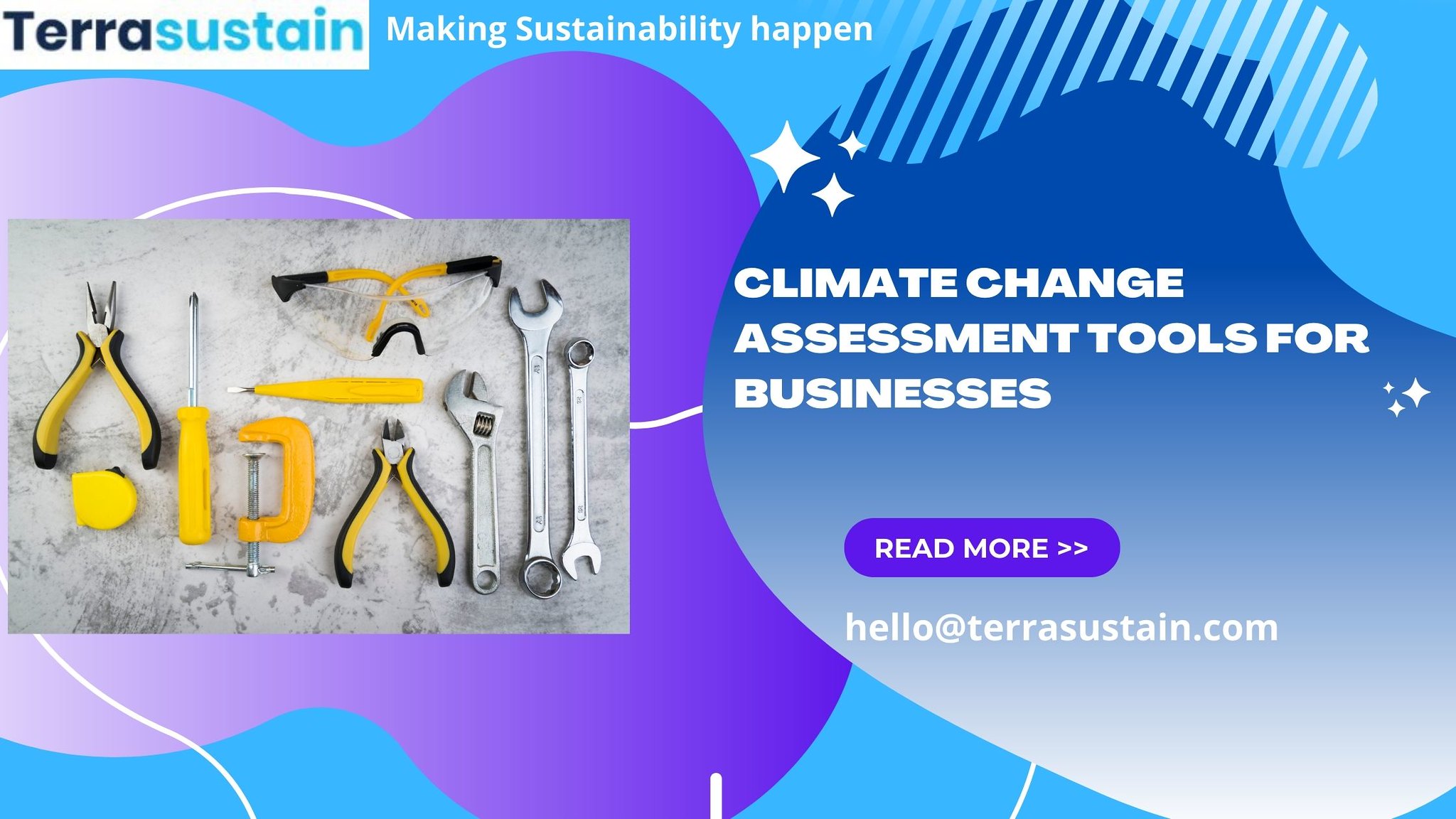The advertisement for Terra Sustain features a visually striking and digitally designed rectangular image, centered around their slogan "Making Sustainability Happen." The background is a light blue gradient adorned with vibrant swirls and engaging graphics, including a purple blob on the left and a blue bean shape on the right, peppered with white four-point stars and lines, adding an elegant touch.

On the upper left, a white area contains the company's name, "Terra Sustain," in black and blue letters. To the right, also in white, the slogan "Making Sustainability Happen" is prominently displayed. In the center, over the blue bean shape, bold white uppercase letters declare: "Climate Change Assessment Tools for Businesses."

A photograph overlays the purple blob on the left, showcasing a variety of mechanic tools with yellow handles, including wrenches and safety glasses, indicating the practical tools Terra Sustain offers to assist businesses. Just below, a purple button labeled "Read More" suggests further exploration, guiding viewers to click for additional information. Beneath this button is the contact detail, "hello@terrasustain.com," all in white, providing a direct link to the company's resources. This dynamic and colorful advertisement effectively captures attention while conveying essential information about Terra Sustain's climate change assessment tools for businesses.